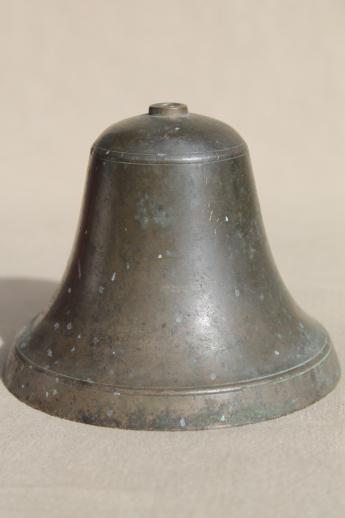This image features a single, old and worn-out bell made of heavy metal, likely brass. The bell is positioned on a neutral beige carpet. The bell, lacking any attachments or decorative elements, has a rough, textured surface with signs of age such as dents, scratches, and areas of rust and corrosion. Its predominantly grayish color is interspersed with patches of beige, brown, and lighter white spots, indicative of oxidation. A distinct band encircles the bottom, and the oxidation appears more concentrated on the left side. The top of the bell has a small lip where a loop may have once been screwed in for hanging. The bell casts a shadow to its left, and despite reflecting light in some areas, the surface is not well polished, emphasizing its historical and unrefined appearance.